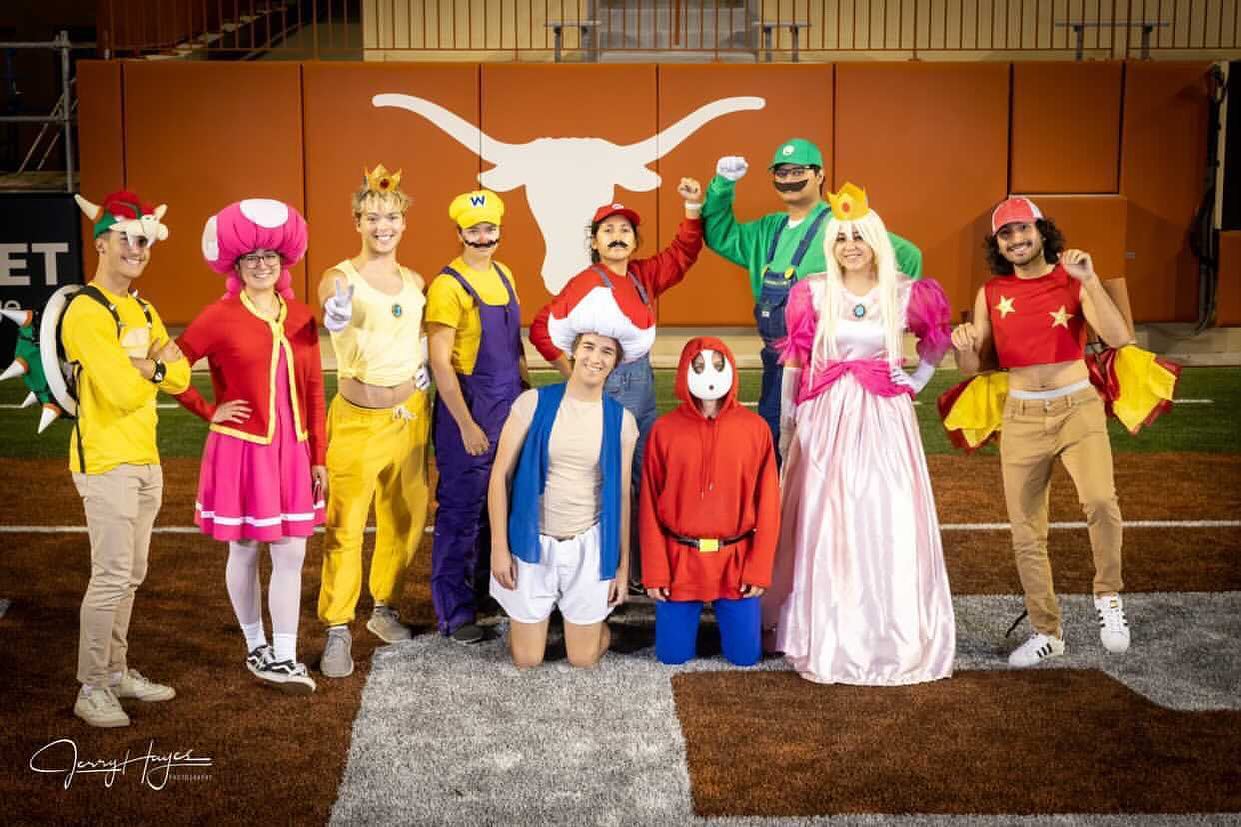This color photograph captures a vibrant indoor scene featuring a group of teenagers, all dressed as iconic characters from the Super Mario video game series, posing against an orange backdrop adorned with a white silhouette of a Longhorn cattle head and the label "Jerry Hayes Photographer." The setting includes a brown and gray carpet or rug atop a surface that resembles turf tinted orange and white.

From left to right, the characters include:

- A young man as Bowser, wearing khaki pants, a long sleeve yellow shirt, white sneakers, a backpack shaped like Bowser's spiked shell, and a hat resembling Bowser's face.
- A woman dressed as Toadette, featuring a pink dress, a red sweater, white socks with black sneakers, and a large pink-and-white polka dot mushroom hat.
- A man portraying Princess Daisy, in a yellow cropped tank top, yellow pants, and gray sneakers, complete with a crown.
- Another individual as Wario, outfitted in purple overalls, a yellow shirt, yellow hat, and sporting a mustache.
- A woman as Mario, visible from the top only, donning a red shirt, red cap, and a mustache.
- A person dressed as Toad, kneeling in front, wearing white shorts, a beige shirt, a blue vest, and a mushroom cap.
- Another person kneeling beside, dressed in a red hoodie, blue pants, and a white mask.
- In the back row, a man as Luigi stands tall with his green shirt, coveralls, green cap, and a mustache.
- In front of Luigi, a woman dressed as Princess Peach with a long, shimmering pink gown, blonde wig, and a crown.
- Finally, on the far right, a man dressed as Ash Ketchum, in a red cropped tank top with yellow stars, brown pants, white sneakers, and a red hat.

The photo exudes a sense of joy and creativity, as each individual brings their respective video game character to life with thoughtfully designed costumes.